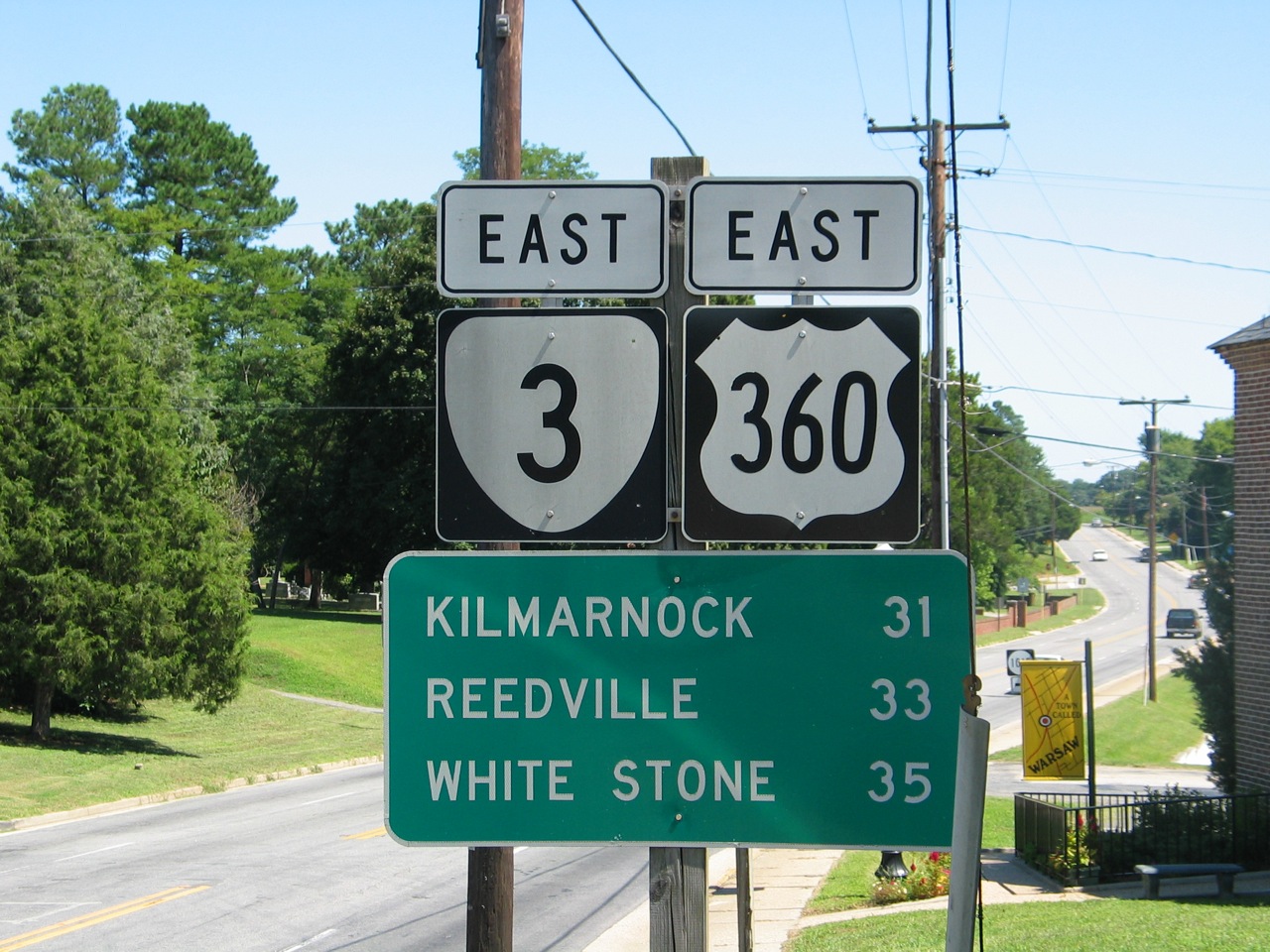This daytime photograph captures a roadside scene featuring a prominent green highway sign with a white border, displaying travel distances to nearby towns. The sign indicates that Kilmarnock is 31 miles away, Reedville is 33 miles away, and White Stone is 35 miles away. Directly above this information are two black highway markers with white ovals: the one on the left signifies East Highway 3 with a bold "3," while the one on the right indicates East Highway 360. The image also includes elements of the surrounding area. On the right side of the road, a building and a black fence enclosing plants with green leaves and red flowers are visible. Across the street, there is a four-lane road with two lanes in each direction. The background showcases a quiet residential street with only two cars visible in the distance, flanked by well-maintained green lawns and lush, full trees, suggesting it is likely around noon.